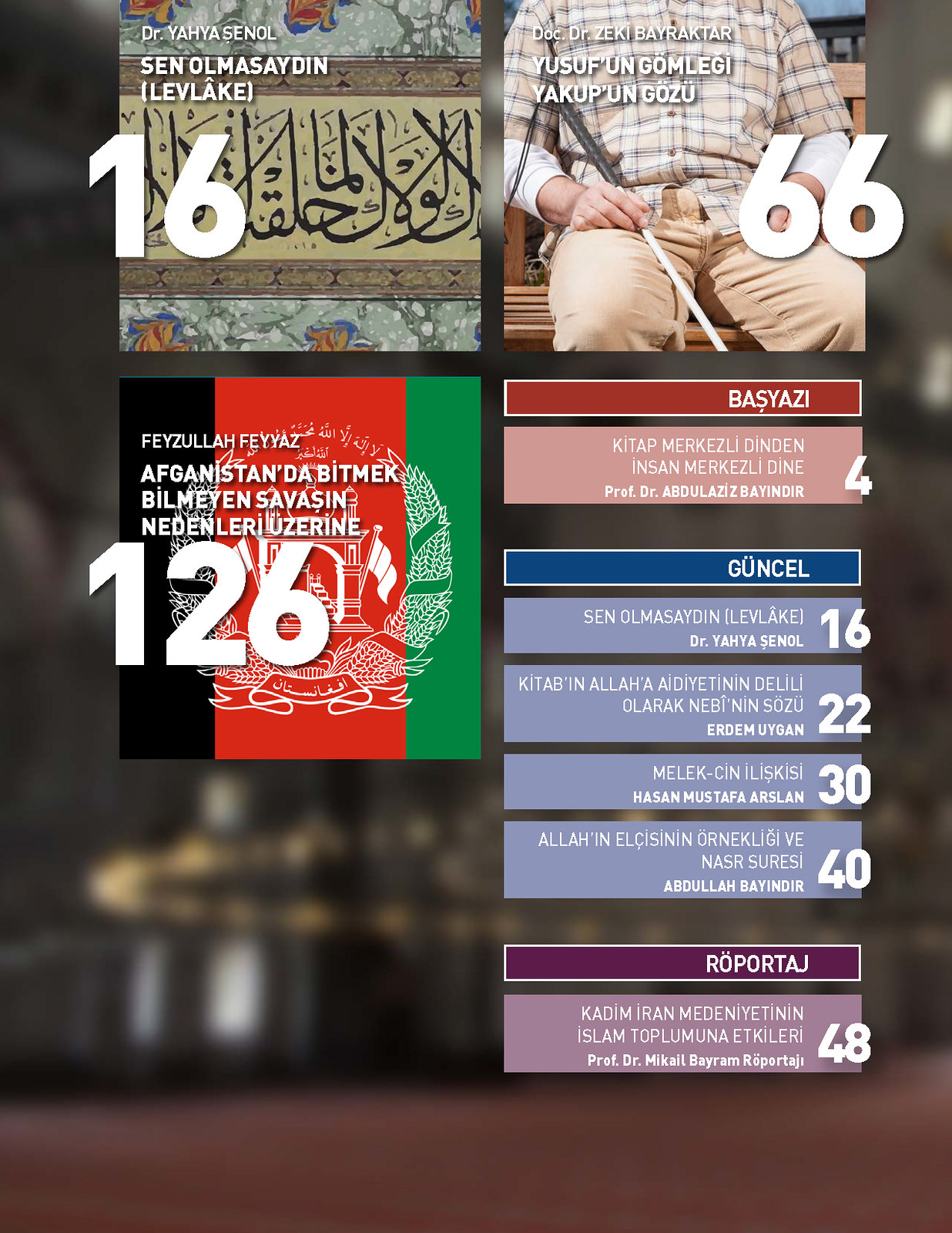The color image is a vibrant advertisement featuring various elements and a range of colors including black, white, red, green, blue, purple, brown, and beige. The background is a blurred photograph with dark gray and purple-red tones. Three large squares with white numerals dominate the layout, each presenting different imagery. The top-left square shows an Arabic script photograph alongside the number 16. The adjacent square features a man in a light brown button-down shirt holding a white cane used by the visually impaired, paired with the number 66. The third large square displays a flag with black, red, and green stripes, marked by the number 126. Smaller rectangles scattered across the layout contain foreign script and numbers. One rectangle bears the number 4, while a group of four blue rectangles display the numbers 16, 22, 30, and 40. Positioned at the bottom right, a single purple rectangle is numbered 48. The text throughout the image includes phrases like "Doc, Dr. Zeki Bayraktar" in Turkish or another language, amidst an overall bright and clear composition.